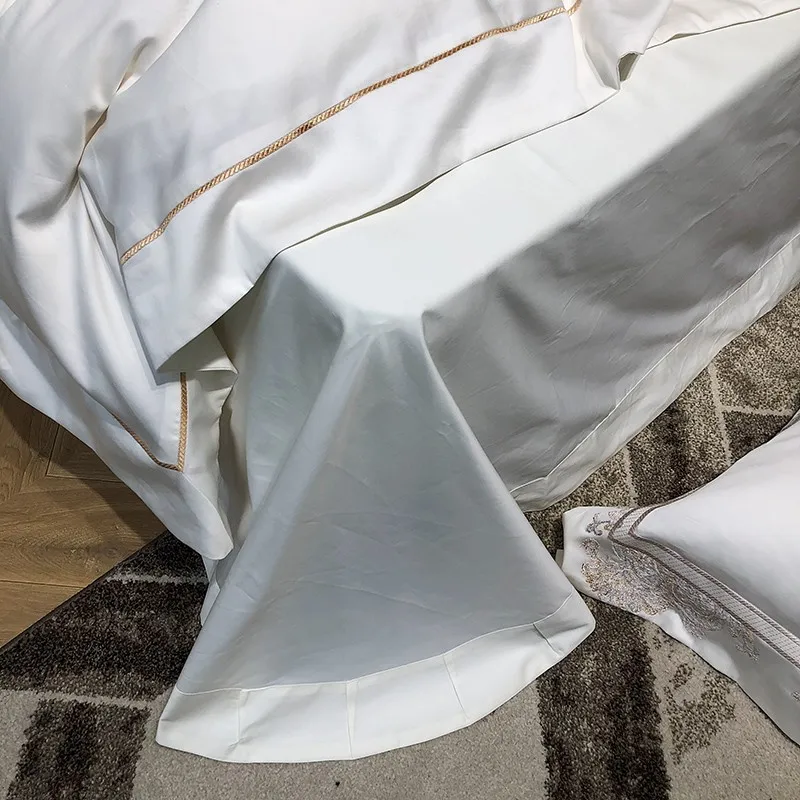A cozy bedroom corner features a luxurious bed with satin white sheets, meticulously adorned with a gold braided trim approximately three inches from the edge. The bed, modestly elevated less than a foot from the hardwood floor, exudes an understated elegance. Beneath the bed, a throw rug in hues of brown, gray, and tan adds a subtle warmth to the space. A single throw pillow, sporting an intricate bronzy gold pattern, lies artfully on the floor, further elevating the room’s opulent ambiance. The top sheet and pillows are neatly covered, enhancing the overall refined aesthetic of this inviting sanctuary.